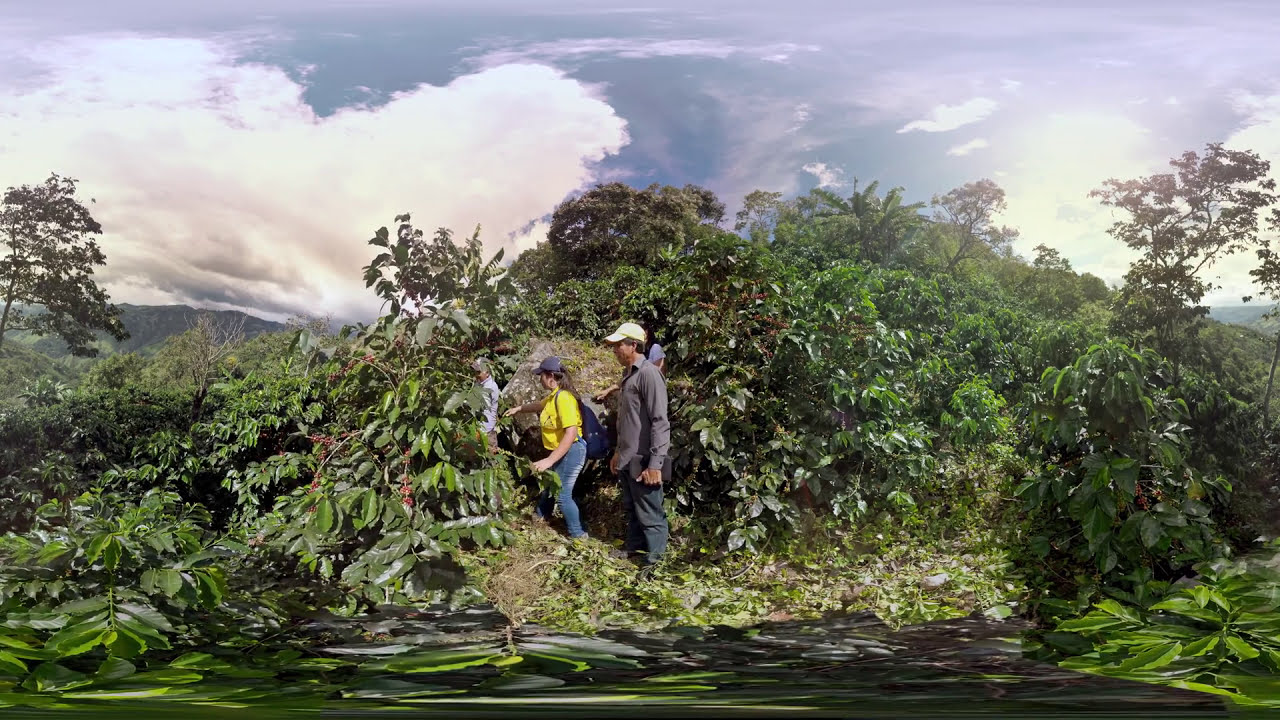In the image, three people are depicted standing amidst a dense, green foliage area, which resembles a jungle or thick brushland. Central to the scene, a man in a light gray shirt and dark pants stands, looking to his left. Beside him, a woman with a ponytail through her hat wears a yellow shirt and blue jeans. The third person, partially obscured by the thick greenery, wears a blue shirt and a gray hat. They all seem to be cutting through the lush vegetation, possibly following someone. A small body of water is visible towards the bottom of the image, adding to the rich natural setting.

Above them, an overcast sky dominates with prominent clouds, and a mountain is discernible to the left, shrouded by the cloud. Despite the clouds, patches of clear blue sky peek through. The overall scene is vibrant with shades of green from the shrubbery and foliage, contrasted by the colors of their clothing—gray, yellow, blue—and the natural hues of brown and light gray from the environment and sky. This outdoor scene, likely taken in daylight, captures a moment of navigation through nature, surrounded by a lush, verdant landscape.